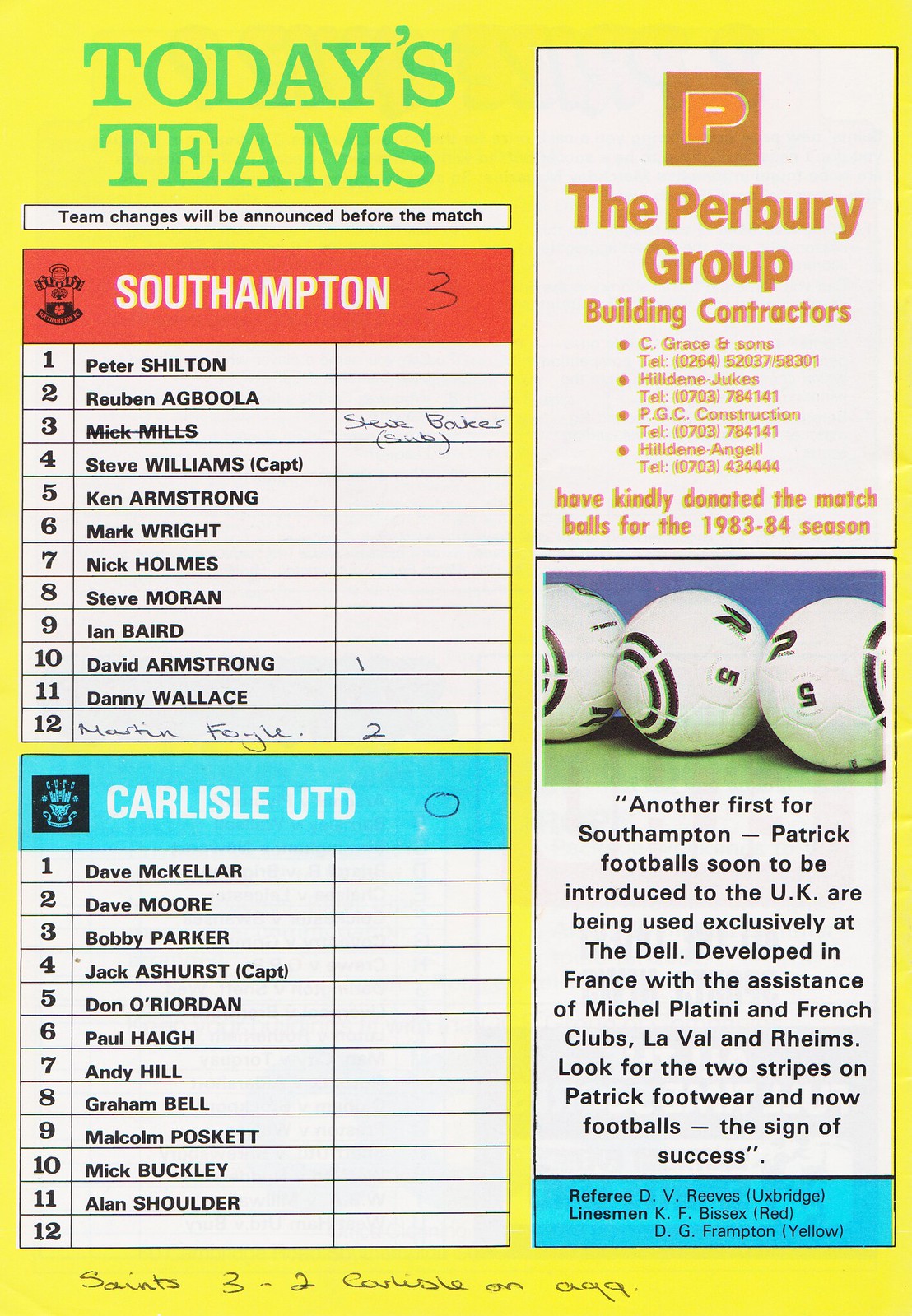The image depicts a detailed player's scorecard for a soccer match, presumably from a game program. The page features a yellow background with "Today's Teams" written in green lettering at the top left. At the top of the page, under a red-bordered section, is the team Southampton, listing 12 players. Below this, in a pale blue-bordered section, is Carlisle UTD, with 11 players listed. The right side of the page contains two advertisements. The first ad, at the top, is for "The Burry Group" building contractors. The ad at the bottom features an image of three soccer balls and announces: "Another first for Southampton - Patrick footballs, soon to be introduced to the UK."